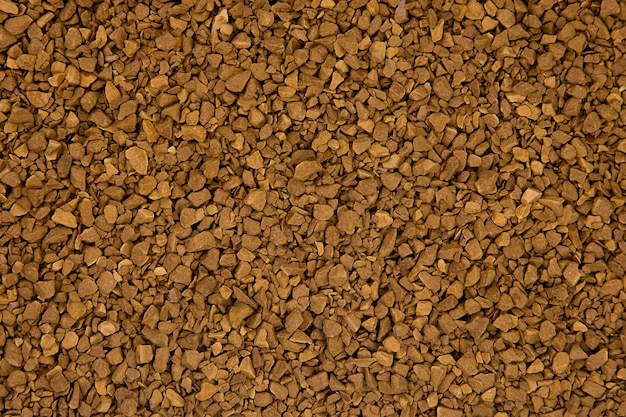The image depicts a vast, uniform expanse of small rocks, pebbles, or gravel, all possessing an orange to brownish hue with some grayish tones. These rocks appear tightly packed together, creating a rough, textured surface that covers the entire view with no other elements like plants, trees, or different rock types present. The pebbles exhibit un-uniform shapes, reminiscent of instant coffee grinds, and are evenly spread out, resulting in a consistent yet varied pattern across the image. Black shadows and gaps between some rocks add depth and contrast to the scene.